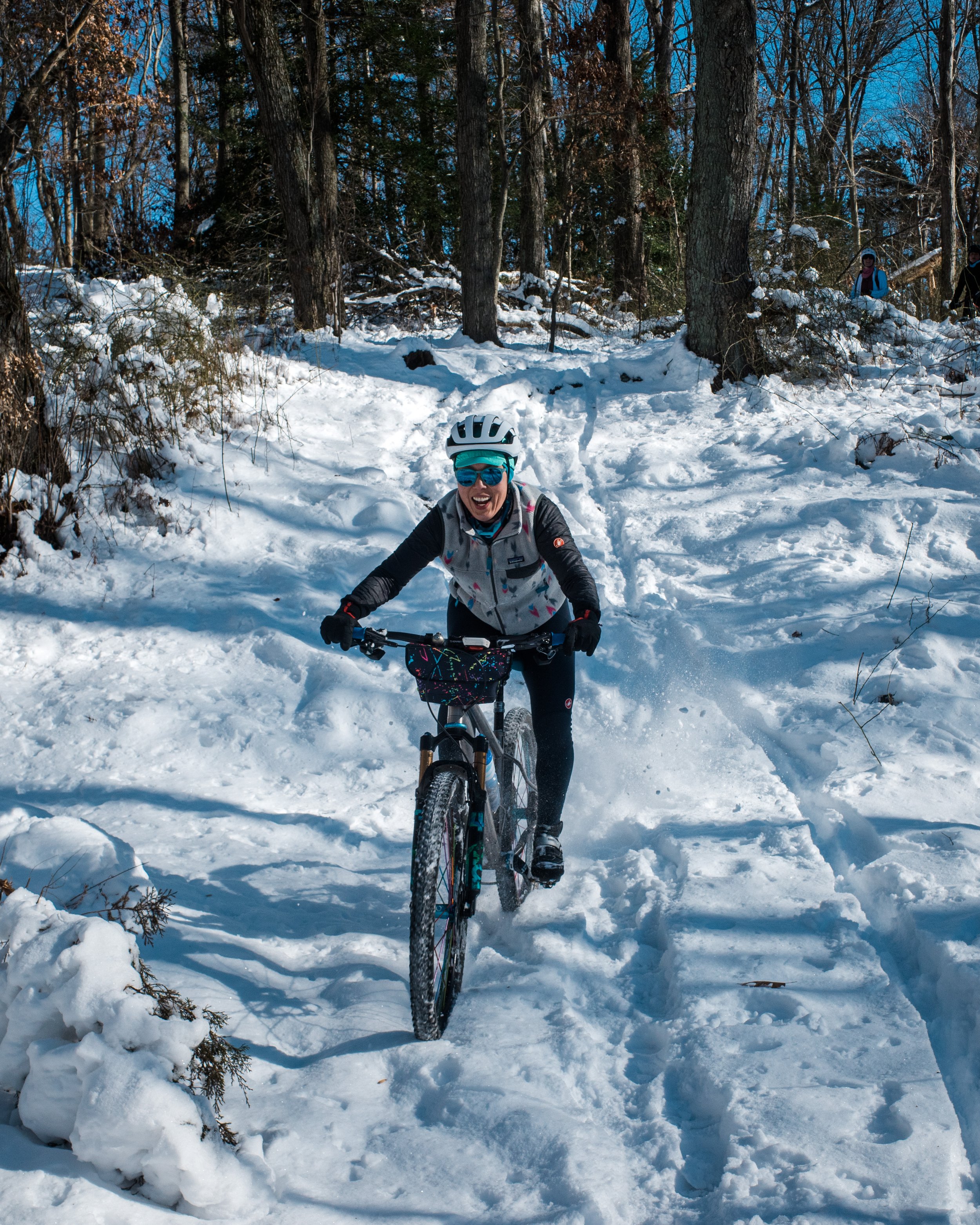The photograph captures a woman riding a mountain bike down a snowy trail in a forest environment. She is centrally positioned, looking directly at the camera with a joyful expression, almost laughing. The snowy path beneath her is white and marked with bike trails, suggesting she has already traveled some distance. The woman is dressed in a predominantly black outfit, complemented by a white vest and a turquoise or blue hat peeking out from under her white helmet. She sports green sunglasses, adding a splash of color to her attire. Her mountain bike is gray with black tires, designed for off-road conditions. In the background, the sky is a clear blue, contrasting with the dark, leafless trees which stand tall with strong, brown trunks. There are also bushes to her right, blanketed in snow. Additionally, another individual appears in the distance, either walking or biking along the snowy trail. The overall scene is a picturesque winter day, filled with the serene beauty of bare trees and crisp, white snow.